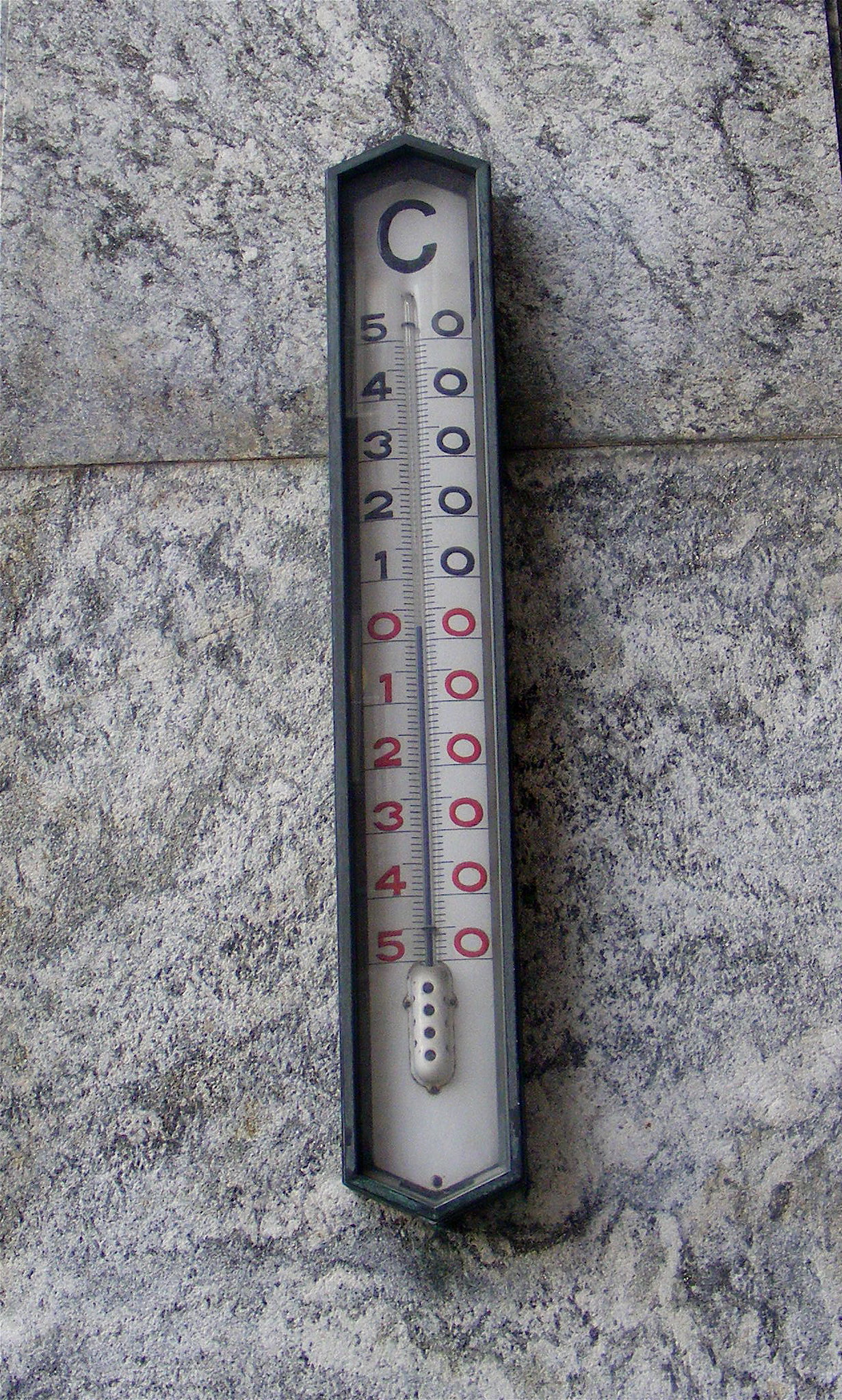An old, cylindrical thermometer is prominently featured against a textured stone surface, which displays a mesmerizing blend of light gray and grayish-blue hues in an abstract pattern, reminiscent of natural rock formations. The thermometer is encased in a protective half-cylinder with a white background, allowing the numerical markings to stand out clearly. Down the middle of the thermometer runs a thin line for the mercury, indicating the temperature in degrees Celsius. The scale is marked with temperatures in increments of ten, ranging from -50°C at the top to 50°C at the bottom. Each interval is clearly labeled, ensuring precise readings. At the very bottom, a small cylindrical reservoir houses the mercury, ready to reflect the current temperature.